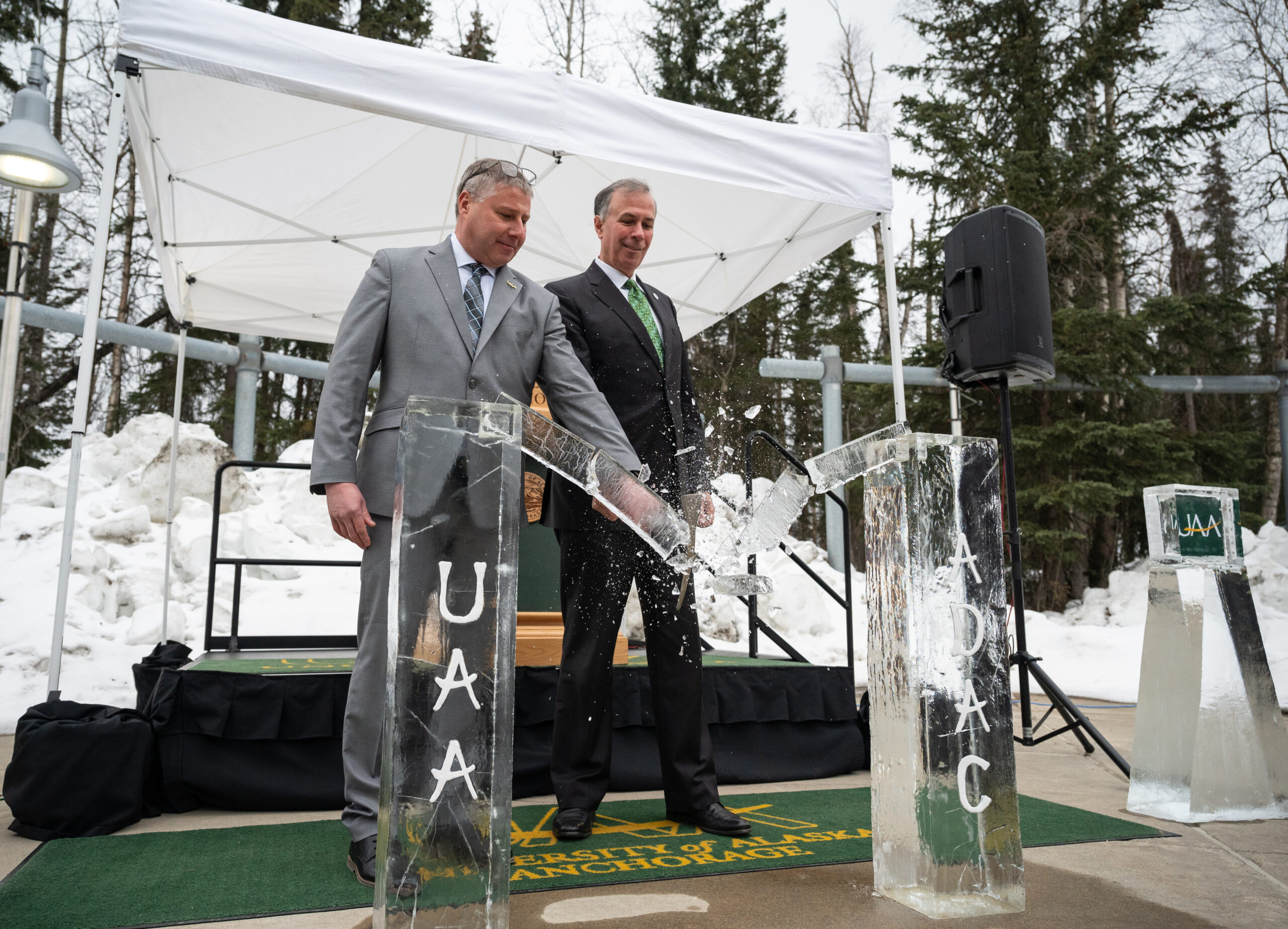This photograph captures a ceremonial moment involving two middle-aged men, both dressed in three-piece suits, participating in an unconventional ribbon-cutting event. Instead of a ribbon, they are shattering a bridge-like piece of ice or possibly a clear material such as glass or lucite. The ice bridge is supported by two waist-high pillars, each bearing inscriptions – one reads "UAA" and the other "ADAC." The man executing the smashing is in a light gray suit with a blue tie, and he has reading glasses perched on his forehead. His counterpart, standing close by, is dressed in a charcoal suit with a green tie.

Both men are smiling and focused on the task at hand. The setting is outdoors, amidst a mountainous, wooded area with numerous pine trees and snow banks, suggesting it's winter. The scene takes place on a green carpet that has "University of Alaska, Anchorage" written in yellow letters, laid in front of a small stage or platform area also surrounded by snow piles. A speaker system is visible, implying the event is being recorded or broadcasted.